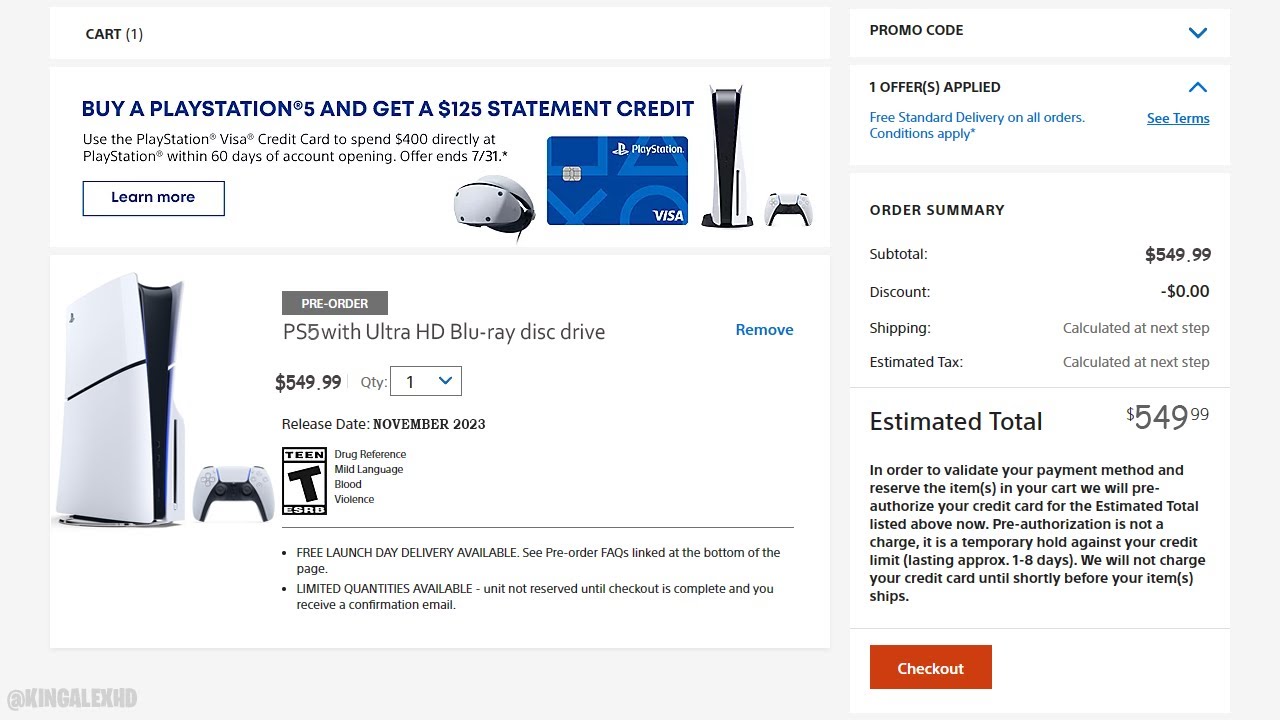The image is a screen capture of the PlayStation website. In the upper left corner, it shows "Cart (1)". Below that, there's a promotional banner stating: "Buy a PlayStation and get a $125 statement credit." The offer details specify: "Use the PlayStation Visa Credit Card to spend $400 directly at PlayStation within 60 days of account opening. Offer ends 7-31." A "Learn More" link is present below these details.

To the right, there are images showcasing the PlayStation VR, a PlayStation Visa credit card, a PS5, and a PS5 controller. Below these images, there is another image featuring a white PS5 console paired with a white PS5 controller, accompanied by the text: "Pre-order PS5 with Ultra HD Blu-ray Disc Drive." A blue "Remove" button is positioned to the right.

Further down, it indicates the price as $549.99, quantity of 1, release date in November 2023, and the product rating as "T for Teen". On the right side of the screen, there's a promo code drop-down menu. Below that, it mentions: "One offer applied: Free standard delivery on all orders (conditions apply, see terms)." 

The "Order Summary" section lists:
- Subtotal: $549.99
- Discount: $0.00
- Shipping: Calculated at next step
- Estimated Tax: Calculated at next step
- Estimated Total: $549.99

At the very bottom, there is an orange "Checkout" button.